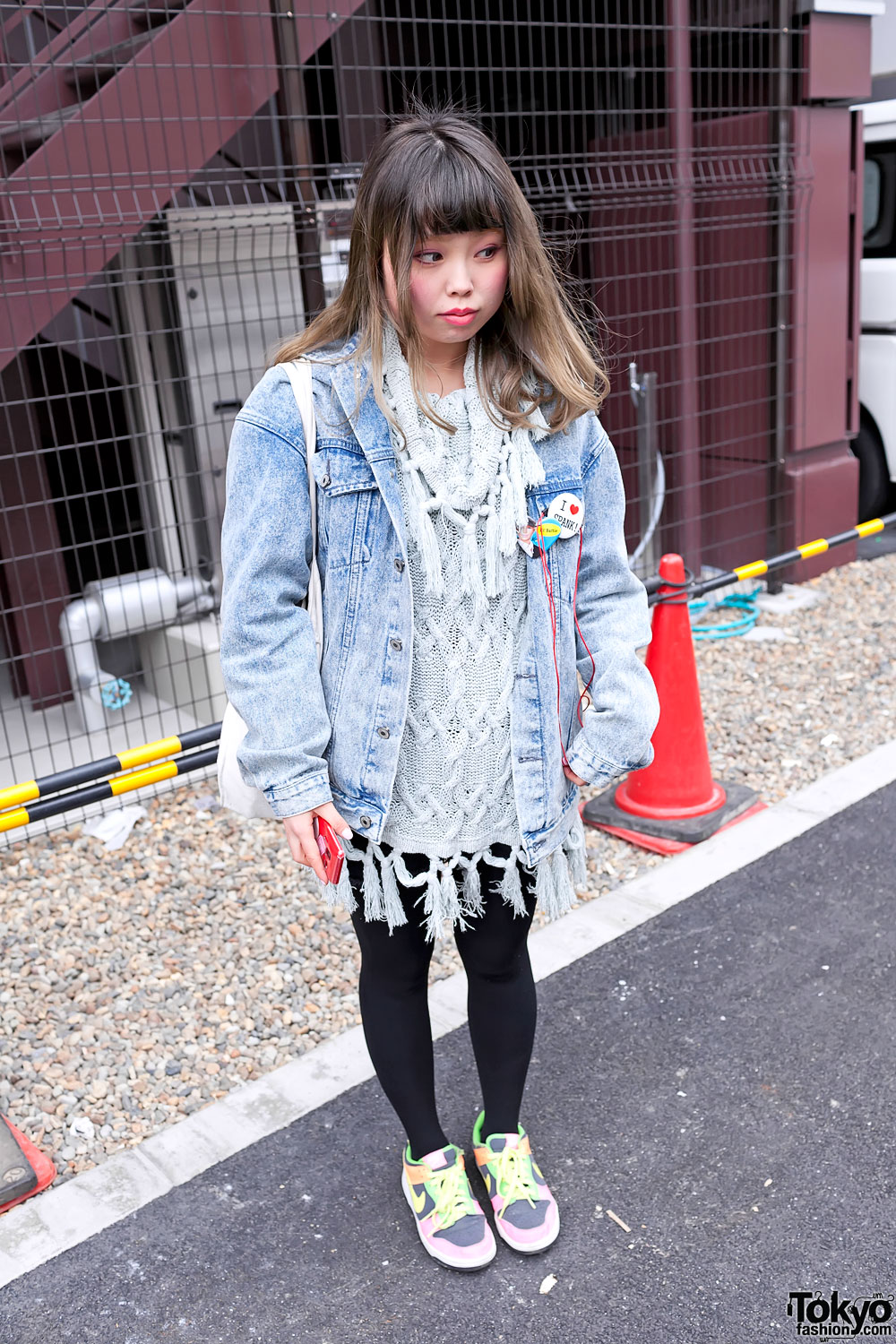The image features a fashionable young Asian woman standing on a black pavement street in front of a curb. She has shoulder-length brown hair with balayage, transitioning to a lighter shade towards the tips, and she sports bangs. She wears makeup, including pinkish-red lipstick and rosy cheeks, with her eyes glancing to her left while her face is slightly forward, giving a smirk-like expression. She's dressed in a grey knit sweater with fringes at the top and bottom, layered under a denim jacket adorned with pins—one of which reads "I love spark." She pairs this with black leggings and multicolored Nike shoes featuring highlighter green and pink accents. She holds a red smartphone in her right hand and carries a white purse on her right shoulder. Behind her are landscaping rocks, black-and-yellow striped pipes aligned above traffic cones, and a rust-colored metal building enclosed with chicken wire fencing, featuring a visible staircase in the upper left-hand corner. A small part of a white vehicle is barely visible in the upper right-hand corner. The lower right-hand corner of the image is marked with the text "tokyofashion.com".